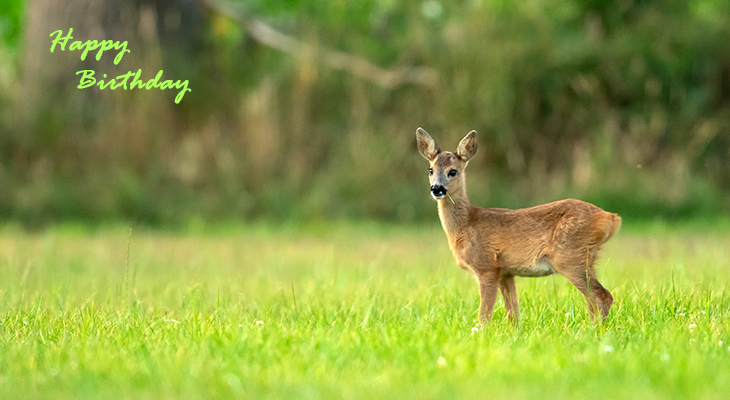In the photograph, a young, juvenile deer stands gracefully in the right side of a lush, green grassy field. The deer, a rich brown color with a white stomach and a grey patch on its otherwise black nose, gazes forward with large black eyes. Its big, triangular ears are also facing forward, giving it a curious yet cautious appearance. The background of the image is beautifully blurred, showcasing the indistinct forms of trees and vegetation, suggesting a wild, untouched setting. On the upper left corner of the photo, a cheerful “Happy Birthday” message is scripted in green cursive text. The deer’s legs are hidden by the tall grass, emphasizing its small size and youthful delicacy, while the lack of other animals around highlights its solitary presence in this serene environment. A small piece of grass is visible in its mouth, adding to the idyllic and innocent nature of the scene.